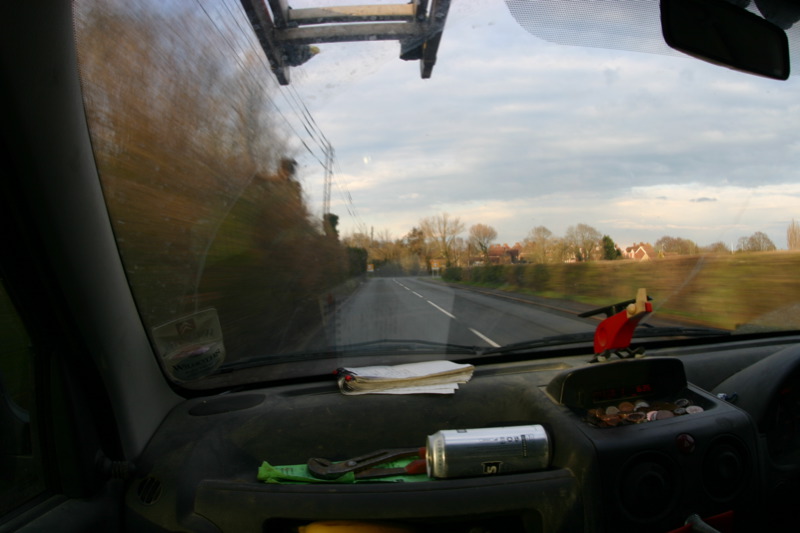The image captures a detailed view from inside a work vehicle, possibly a truck or van, while driving on a countryside road. The interior of the vehicle reveals a cluttered dashboard with various items. On the right side, there is a tray filled with numerous coins. Adjacent to this, in the dashboard groove, rests a silver aluminum beverage can and a pair of pliers. Additionally, a small green notebook or notepad is visible, lying on top of the dashboard. 

Looking through the windshield, one can see a typical two-lane road with no traffic ahead and blurry trees on the left, indicating the vehicle is in motion. On the right, there is a grassy field lined with bushes and scattered trees, and houses are discernible in the distance. Above the windshield, the tip of an aluminum ladder protrudes, suggesting it is secured on the top of the vehicle. The scene is under a gray, overcast sky filled with clouds, enhancing the feeling of a serene journey through the countryside. The vehicle appears to be right-hand drive, following the left-side path of the road, implying the location might be in a region where left-hand driving is customary.